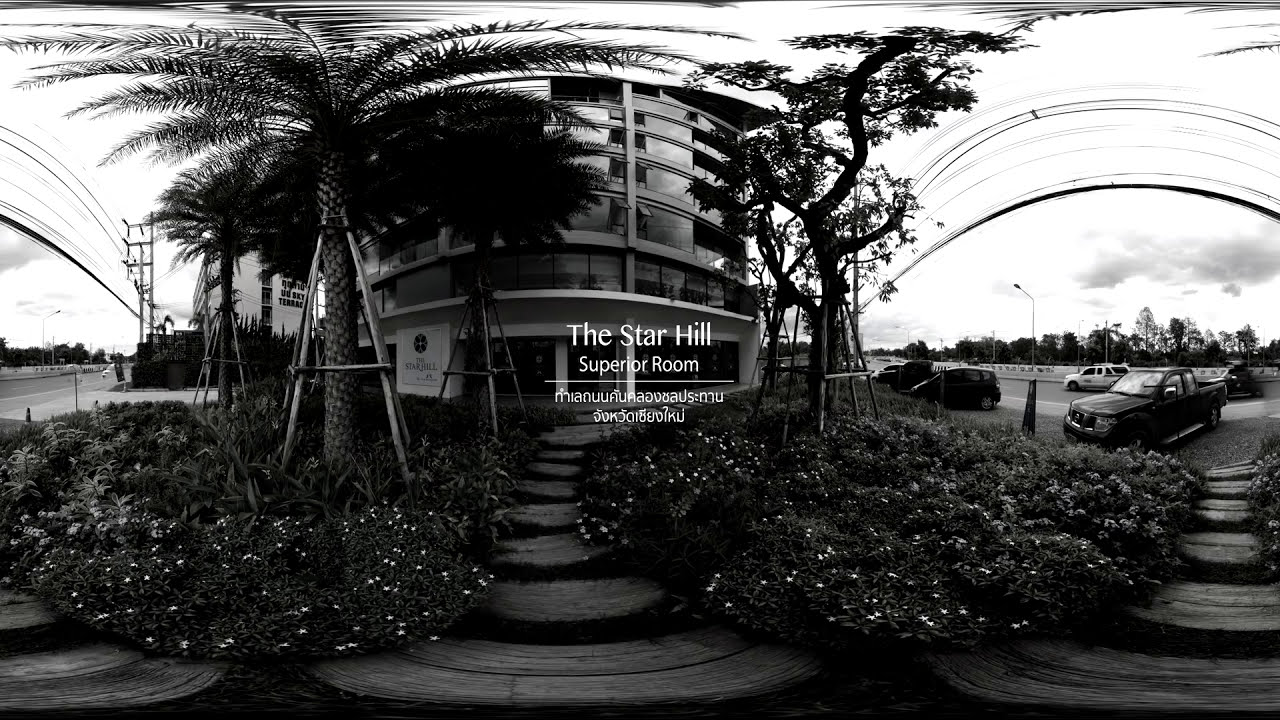The image is a fisheye lens photograph taken during the daytime, showcasing an event center or hotel named "Star Hills Superior Room," as indicated by the text overlay with some foreign language text. The building is approximately six or seven stories tall and light in color. The foreground features a staircase leading to the entrance, flanked by two sections of decorative plants, including bushes with flowers, and palm trees—one supported by sticks. The right side reveals a parking lot with various vehicles, including trucks and cars, and utility poles with lines. The left side displays another building, streetlights, a road, and a fire hydrant. The sky is cloudy, and the image is in grayscale.